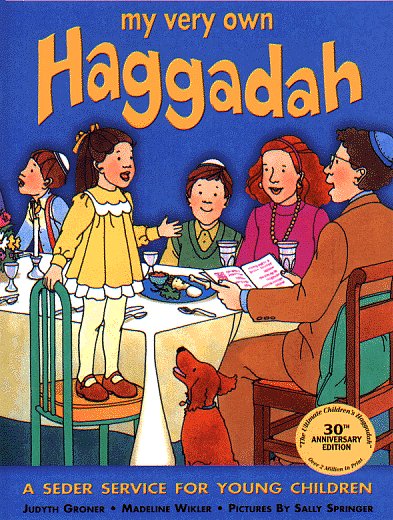The cover of this vertical, rectangular book features a lively family dining scene against a blue background. Central to the image is a dining table covered with a white tablecloth, set with silverware, glasses, and plates of food. Gathered around the table are various family members: a little girl in a yellow dress and brown shoes standing on a chair, a boy in a blue shirt with red overalls, a man in a brown suit holding a book, and two other adults, one in a green sweater and the other with bright red hair wearing a purple turtleneck and a necklace. All the men are wearing yarmulkes, indicating a Jewish ceremonial context. A brown dog with an open mouth looks up at the girl from the floor. At the top of the cover, in orange letters, it says "My Very Own Haggadah," followed by "Haggadah" in white. Beneath, in orange print and all caps, it reads "A Seder Service for Young Children." The authors are listed as Judith Groner and Madeline Wickler, with illustrations by Sally Springer. A gold seal in the bottom right corner celebrates this as the "Ultimate Children's Haggadah, 30th Anniversary Edition," indicating over 2 million copies in print. The scene suggests a joyful Seder ceremony, engaging all its participants in the festive tradition.